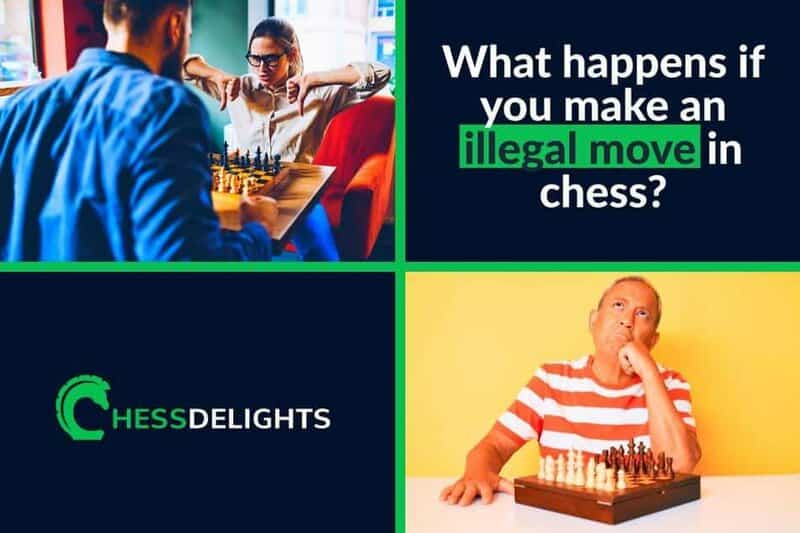The image is a detailed infographic or slideshow about chess, divided into four equally separated sections. 

In the top left section, a man and a woman are engaged in a game of chess. The man is wearing a blue long-sleeved shirt and is leaning towards the chessboard, which is positioned on a white desk. Opposite him, the woman, dressed in a white shirt and glasses, sits in a red chair against a green wall backdrop. She is giving a double thumbs-down gesture, possibly indicating frustration or disapproval. The man’s chess pieces are tan, whereas the woman’s pieces are black.

The top right section features an informative text block. It has a blue background with the phrase "What happens if you make an illegal move in chess?" written in white text. The words "illegal move" are highlighted in green.

In the bottom left section, there is a company logo for "Chess Delights." The word “Chess” is in green with the ‘C’ shaped like a horse chess piece, while “Delights” is in white.

Finally, in the bottom right section, a man in a red and white striped shirt is seated, deep in thought, with his left elbow on the table and his hand resting on his chin. In front of him lies a chessboard with white and brown pieces. His right hand is face down on the white desk, and he appears to be contemplating a move or considering the implications of an illegal move in chess. The backdrop here is a yellow wall.